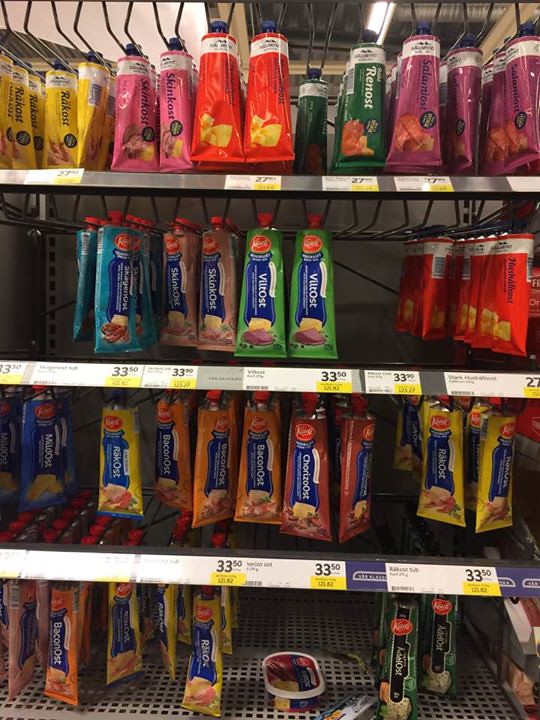The image showcases a section of store shelving, housing neatly organized rows of various colored tubes. There are four shelves in total, each holding tubes suspended from their circular openings at the top. 

On the top shelf, from left to right, the tubes are colored yellow, pink, red, green, and purple. Each is priced at 27 units, though it is not specified whether this is in dollars or another currency.

The second shelf from the top features tubes in colors blue, tan, green, and red, with each priced at $33.50.

The third shelf displays tubes in blue, yellow, light brown, medium brown, and yellow again, all also priced at $33.50.

Finally, the bottom shelf has tubes colored light brown, orange, yellow, and green.

The precise arrangement and clear pricing provide a visually organized view, simplifying comparison and selection for customers.